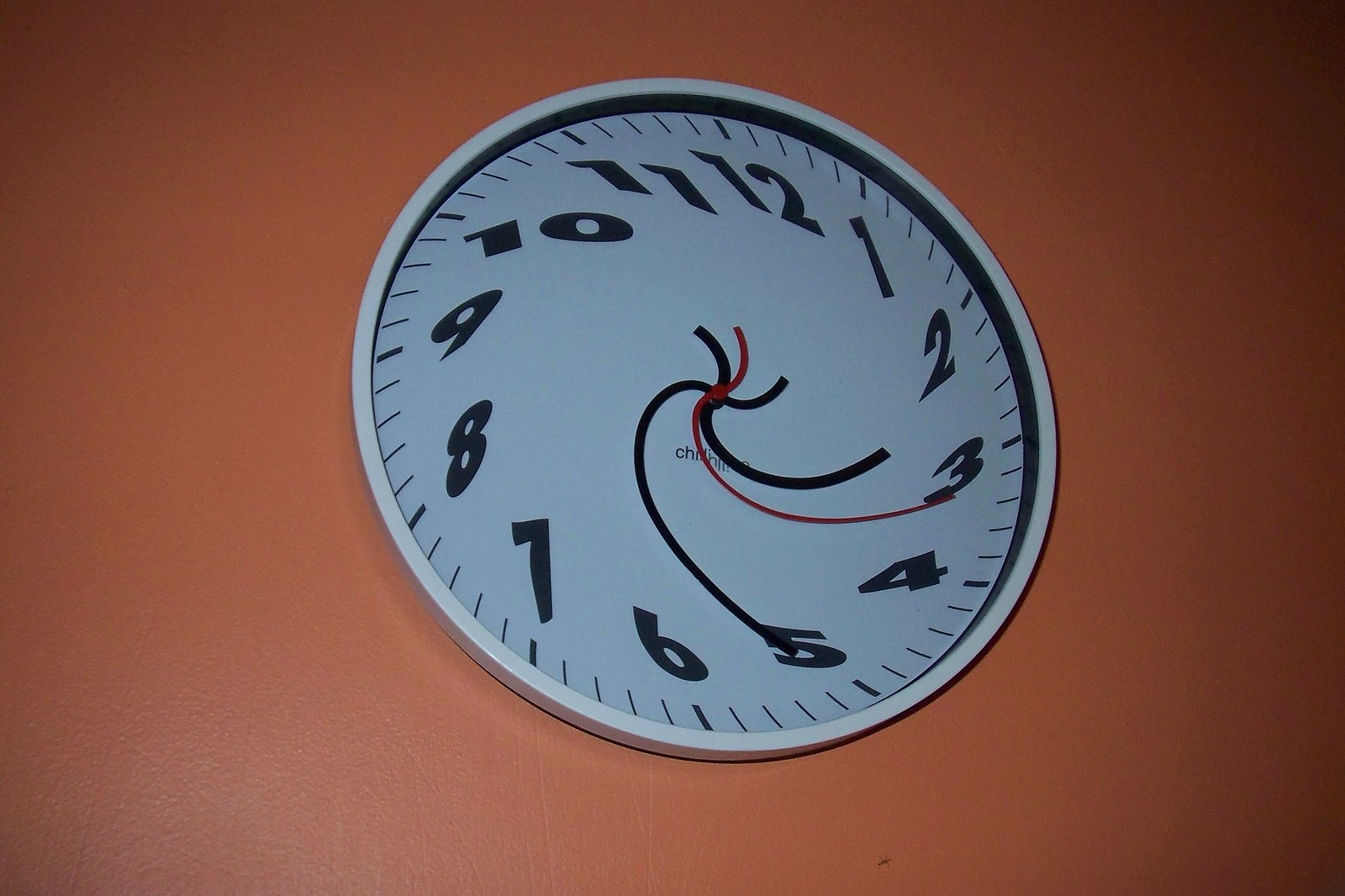In this artistic image, a uniquely distorted clock is the focal point. Set against a rectangular backdrop that transitions from bright orange at the center to a darker, almost coppery hue at the edges, the clock's unusual design immediately captures attention. The clock itself is white with a dual trim of white and black, and its circular face is filled with curvy, swirled numbers arranged around the edge in thick black font. Minute marks also in black ring the clock's face. The hands of the clock add to its eccentricity, with the hour and minute hands being black and the second hand a striking red, positioned at 3, indicating the time 2:25. The overall effect is one of motion and distortion, as if the clock is twisting or being pulled in a circular motion, creating a quirky and eerie visual impact. This image seems to have been manipulated or digitally created to enhance its surreal, artistic style.